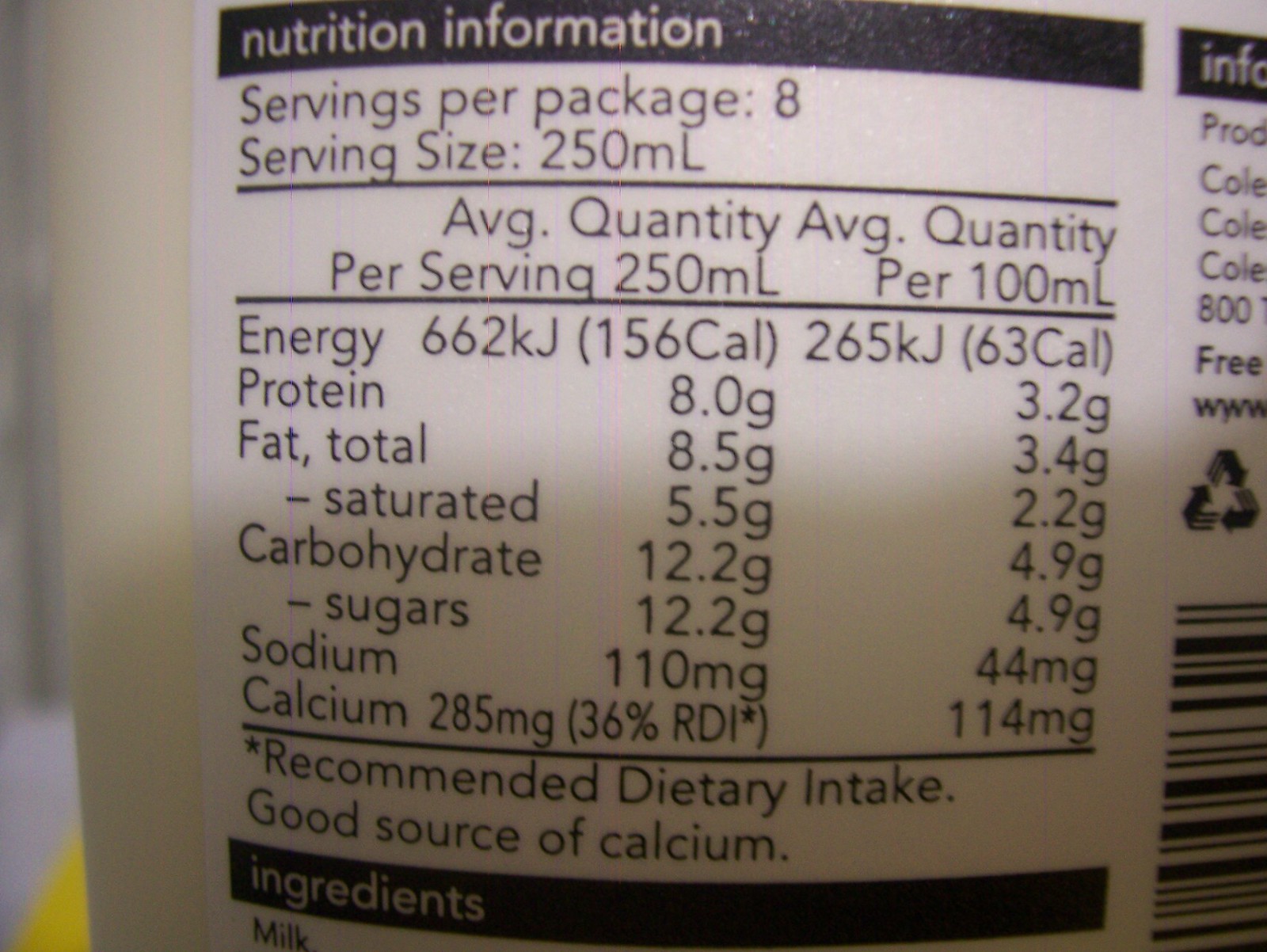Here's a detailed and cleaned-up caption based on the descriptive voice input you provided:

---

The image showcases a detailed view of the nutritional information label on the back of a product. The label is prominently displayed against a surface that appears white and yellow, suggesting it may be resting on a multicolored countertop. The product's name is not visible due to the zoomed-in focus on the label. The upper section of the label has a black header with the phrase "Nutrition Information" written in white text. 

Below this, the label provides serving details: "Servings per package: 8" and "Serving size: 250 mL." A black dividing line follows these details, leading to further nutritional breakdowns. The label specifies the average quantity per serving and per 100 mL, listing values for various nutrients: 

- Energy: 662 kJ
- Protein: 8.0 g
- Total Fat: 8.5 g
- Saturated Fat: 5.5 g
- Carbohydrates: 12.2 g
  - Sugars: 12.2 g
- Sodium: 110 mg
- Calcium: 285 mg

Towards the bottom, highlighted in a separate section, the label notes that the product is a "Good source of calcium," meeting the "Recommended Dietary Intake" guidelines.

---